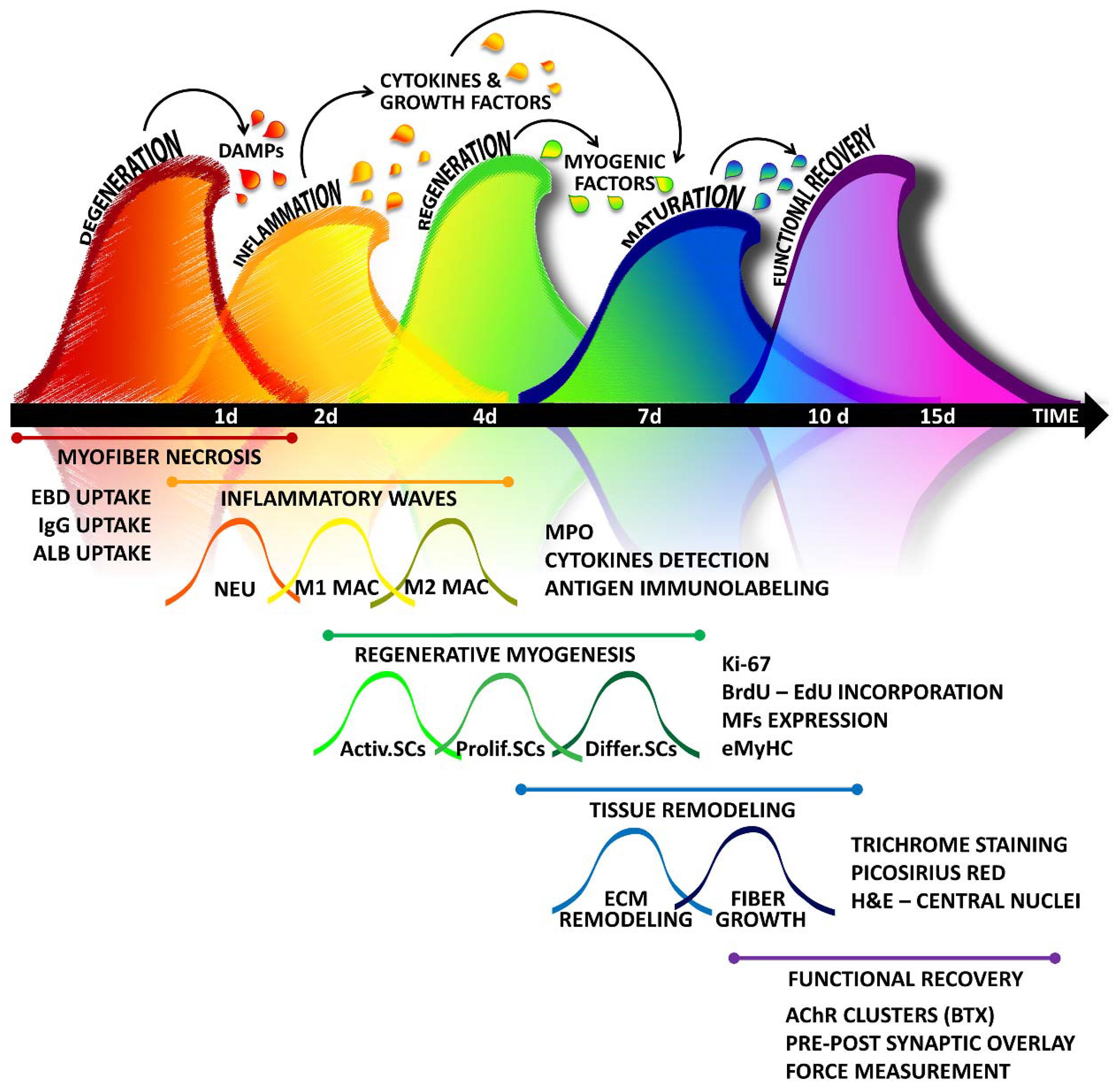The image is a detailed and colorful chart set against a white background, illustrating the phases of myofiber necrosis over a 15-day period. At the center of the image is a black horizontal bar marked with the progressive time points: 1D, 2D, 4D, 7D, 10D, and 15D, followed by the word "time" at the end.

Above this black bar are five distinctive waves shaped like shark fins, each representing a different phase of the process. The first fin is orange and labeled "degeneration," followed by a yellow fin labeled "inflammation." The third fin, representing "regeneration," is green, and the fourth fin, labeled "maturation," blends green and blue. The final fin is violet and purple, indicating "functional recovery."

Beneath the black bar is an additional section of descriptive text, featuring black script over a white backdrop, providing further scientific breakdowns. This text includes references to "inflammatory waves," "regenerative myogenesis," and "tissue remodeling." At the bottom right corner of the image, there is a purple line annotated with "functional recovery," along with terms like "ACHR clusters," "pre-postsynaptic overlay," and "force measurement." This chart visually encapsulates the progression of muscle tissue healing through various biological phases, making it an informative resource for understanding the scientific process involved.